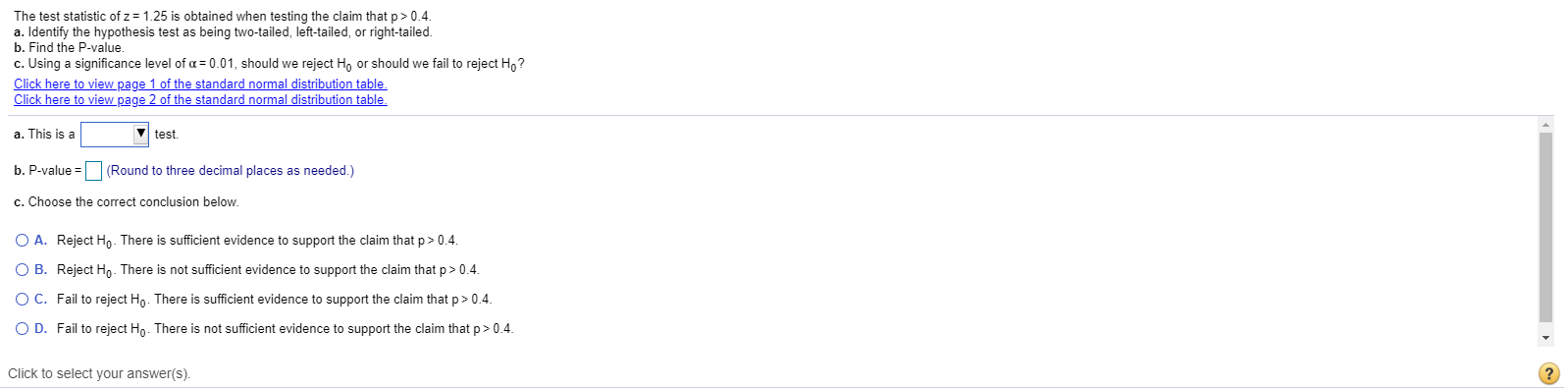This screenshot depicts a survey with multiple questions pertaining to a hypothesis test. At the top, it presents a scenario where a test statistic of Z = 1.25 is calculated to test the claim that P > 0.4. The survey is broken down into several parts:

1. **Identify the Hypothesis Test:** Determine if the hypothesis test is two-tailed, left-tailed, or right-tailed.
2. **Find the P-Value:** Calculate the P-value.
3. **Conclusion Based on Significance Level:** Using a significance level of α = 0.01, decide whether to reject or fail to reject the null hypothesis (H₀).

At the bottom, the survey provides two links highlighted in blue for further reference:
- **Click Here to View Page 1 of the Standard Normal Distribution Table.**
- **Click Here to View Page 2 of the Standard Normal Distribution Table.**

Below these links:
- Under section A: "This is a ___ test." (for entering the test type)
- Under section B: "P-value = ___." (to be rounded to three decimal places)
- Under section C: "Choose the correct conclusion below." This provides four possible conclusions:
   1. Reject H₀: There is sufficient evidence to support the claim that P > 0.4.
   2. Reject H₀: There is not enough evidence to support the claim that P > 0.4.
   3. Fail to reject H₀: There is sufficient evidence to support the claim that P > 0.4.
   4. Fail to reject H₀: There is not enough evidence to support the claim that P > 0.4.

The survey clearly lays out the steps for performing the hypothesis test, from identifying the test type to calculating the P-value and finally, making a conclusion based on the significance level.